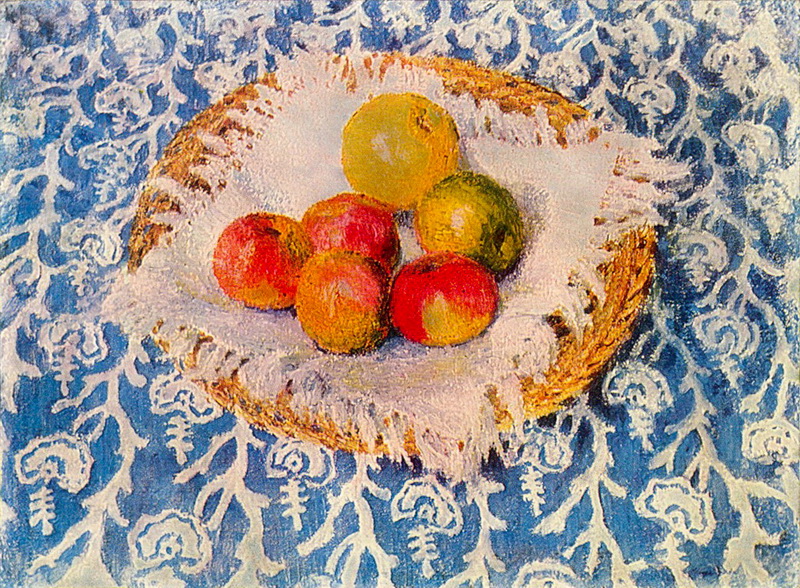This still-life painting features a detailed composition of a wicker plate-like basket holding six apples, four red and two green, positioned on a white fringed napkin. The red apples display lighter spots that are a goldish color, while the green apples have a yellowish tinge. The largest apple, perched on top, stands out significantly in size, almost double that of the others. The basket rests on a blue tablecloth adorned with intricate white floral designs and motifs resembling branches with tiny nubs. The meticulously painted background complements the central arrangement by adding a China blue hue with a white floral pattern, enhancing the overall aesthetic of this vivid still-life scene.